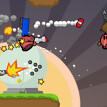This colorful image, likely a small screenshot from a video game, features a dynamic scene with several distinct elements. In the bottom left corner, a bright orange sun illuminates the background, casting alternating light and dark gray sun rays across the composition. Just above a grassy flat hill, a white globe rests on a thin layer of grass. Emanating from this globe, five bullets travel in a V-formation towards the right side of the image, indicated by a yellow flash at the globe's center. A small reddish creature, possibly holding a laser gun, stands with white pants and a pink face. This creature's head is oriented to the left while its feet point to the right, and a trail of four yellow stars follows from its eye. Adding to the vividness are explosion marks and puffs of smoke scattered near the top of the scene, enhancing the chaotic and animated atmosphere.